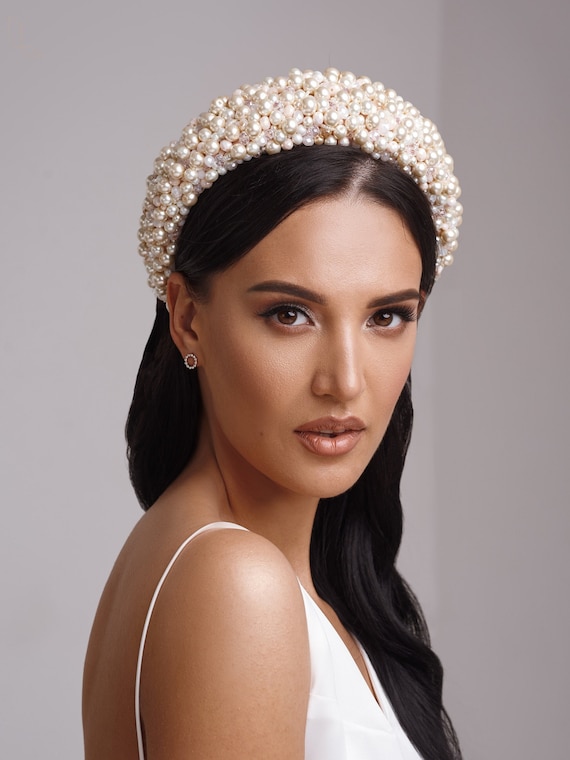The photograph is a detailed portrait in color, oriented vertically. It prominently features a young woman, potentially Middle Eastern, wearing a white, understated V-neck wedding dress with spaghetti straps. The image captures her from the top of her ornate pearl headpiece to about mid-chest. The headpiece is a thick, arched band about an inch and a half wide, composed of pearls in varying shades from pale pink to beige, clustered together to create a crown-like effect.

The woman has long, dark brown hair, parted on the side and elegantly cascading to her left. Her hair also streams down the right side of her face, tucking behind her ears. Her makeup includes nude lipstick and cat eyeliner that accentuates her brick brown eyes. She accessorizes with small, flat diamond circle earrings resting against her earlobes. Captured from a right-side angle, she turns her head slightly back over her shoulder, looking up at the viewer with a subtle, half smile. The background of the image is gray, contributing to the realism and focus on the subject.